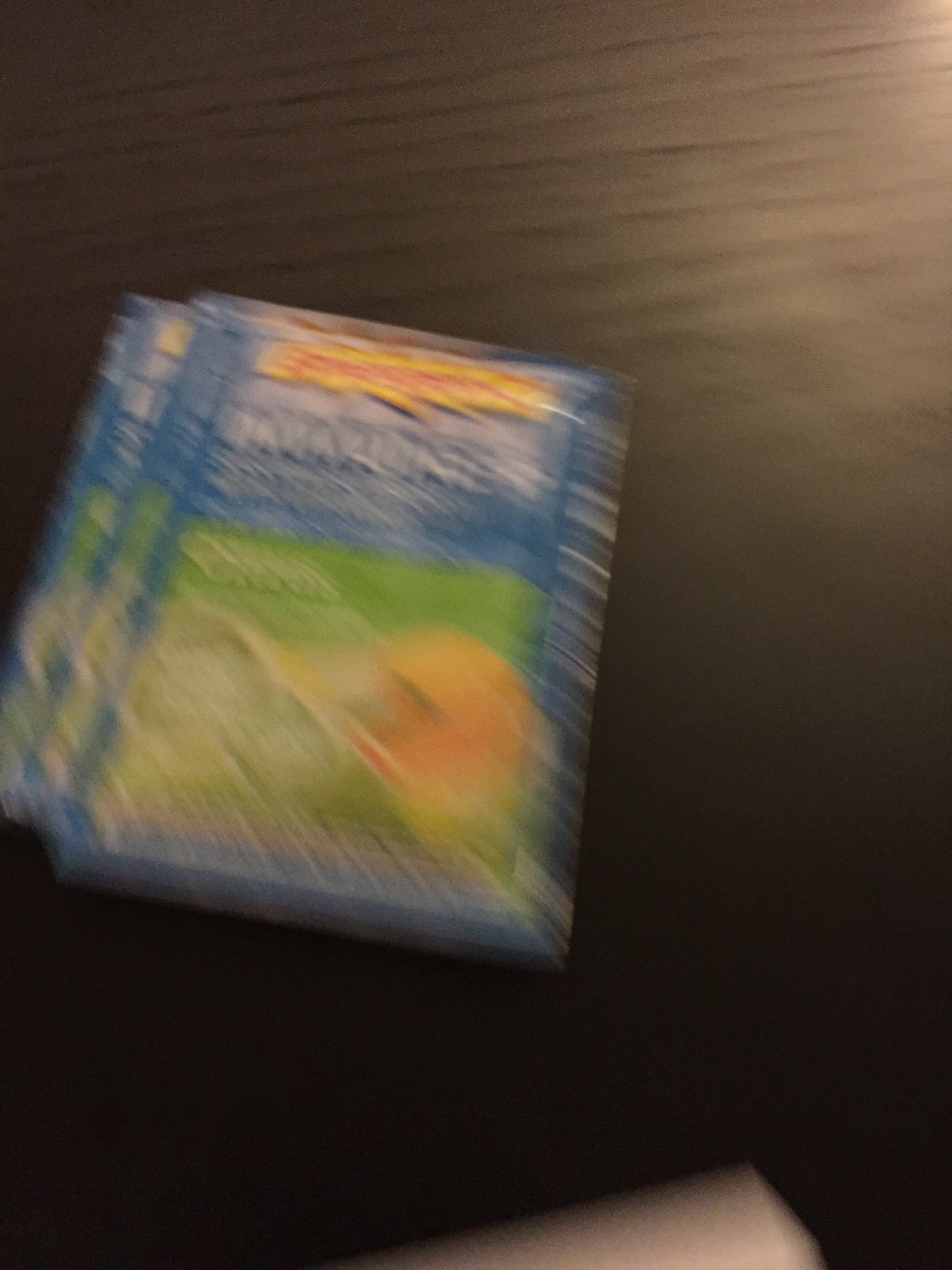This blurry color photograph captures a bird's-eye view of a scene featuring a predominantly brownish wooden surface that gradually darkens towards the bottom. At the very bottom edge, a light brown object, likely a piece of paper or a box, peeks into the frame. Toward the center and slightly to the left, the top of what appears to be a carton is visible. It seems to consist of several similar cartons stacked on top of each other. The carton displays a blue top with some white writing, a yellow section adorned with red text, and a green portion at the bottom which possibly showcases an image of some fruit, perhaps orange or white. Additionally, some white writing on the far right edge of the carton stands out against the blue background.